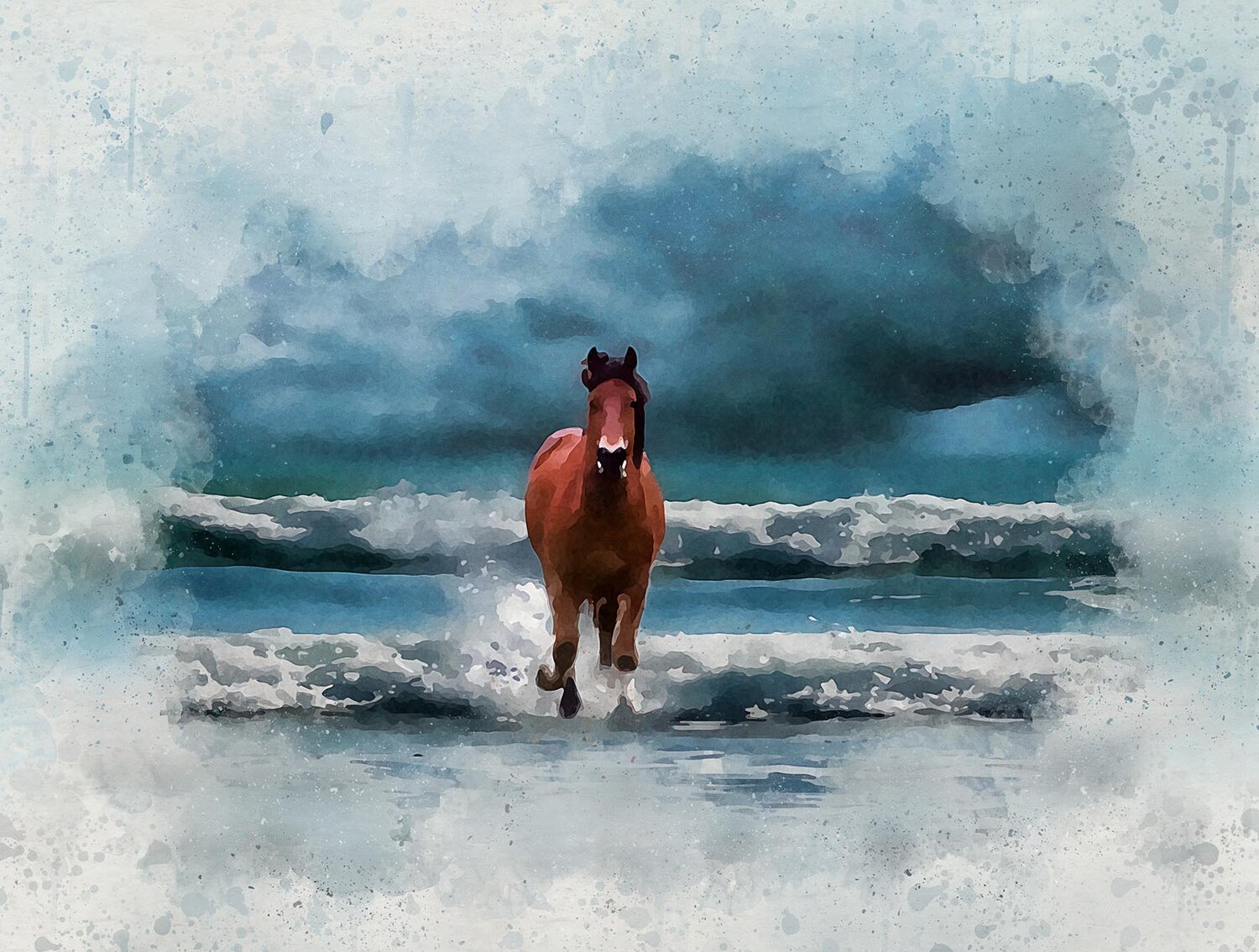This watercolor painting depicts a dynamic scene of a brown horse galloping through the waves. The outer edges of the image feature a faded white vignette, dotted with water droplets that gradually blend into the composition. At the center, a deep blue sky meets equally dark blue water, creating a stark contrast against a large, crashing white wave. Below this, additional stretches of blue water interspersed with white waves frame the horse that charges towards the viewer. The horse, lifting its left leg in a powerful stride, boasts a darker black mane and ears, accented by a distinctive white marking that surrounds its black muzzle. The energy of the scene is palpable as the majestic animal runs through the surf, its form sharply defined against the swirling, foamy water.